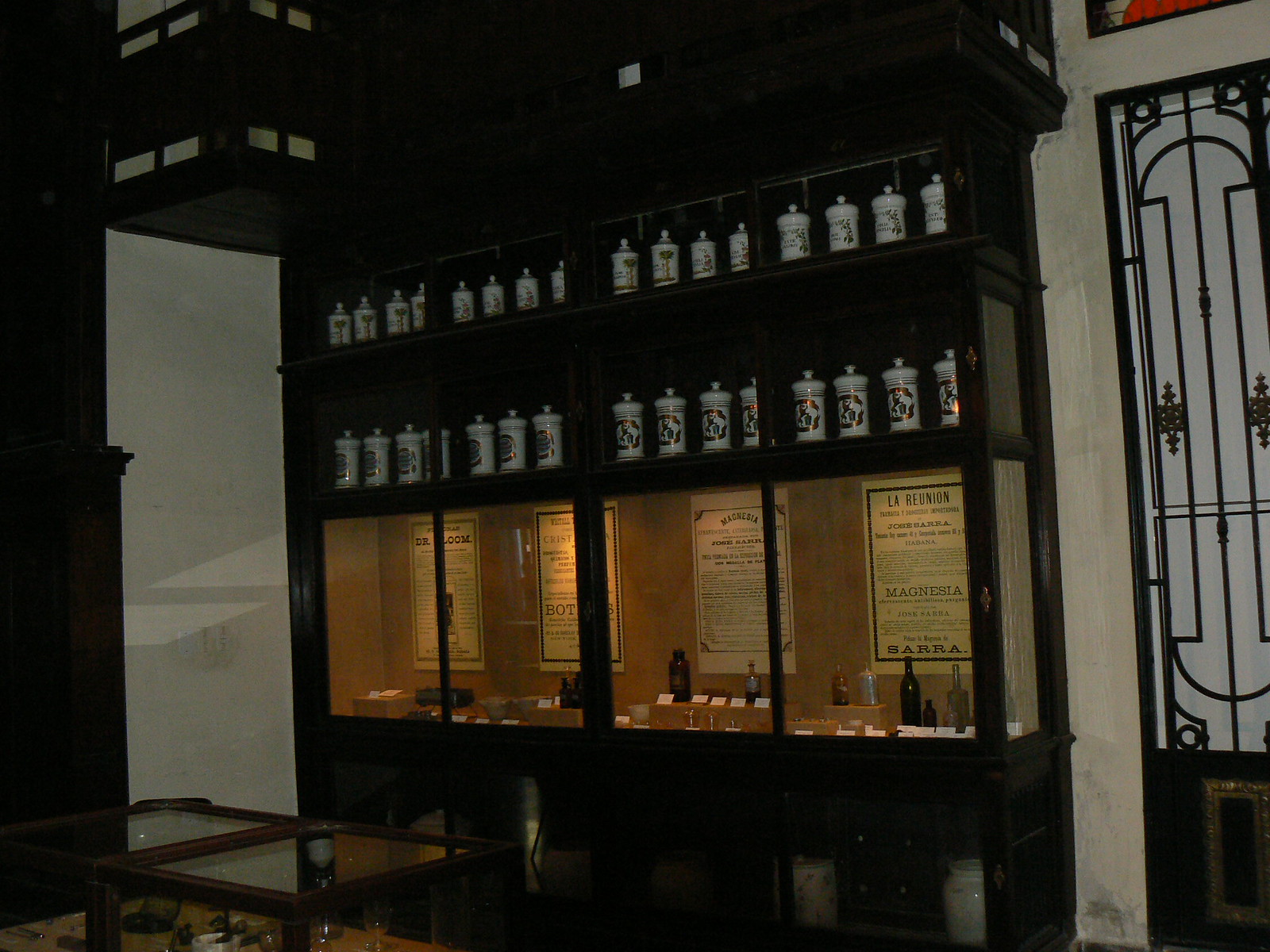The image depicts an interior setting that could be a store or potentially a museum focused on beauty and historical products. The centerpiece is a tall, dark wood armoire divided into four distinct stalls. Each stall is adorned with signs featuring black text on yellow paper, evoking a French feel. These stalls display various beauty products and informational cards that likely detail the items. The overall ambiance of the room is markedly dark, highlighted by the deep wood tones and subdued lighting, contrasting sharply with the room's white walls.

Within the armoire, the upper shelves house white steins with possible red accents, while the lower sections consist of display cases filled with bottles and posters, which might be in Spanish. Additionally, the black shelves and glass cases are accented by internal lighting, drawing attention to the items displayed. A door is positioned to the far right of the scene. The atmosphere suggests a blend of historical reverence and contemporary showcase, whether it's in a retail or educational context.